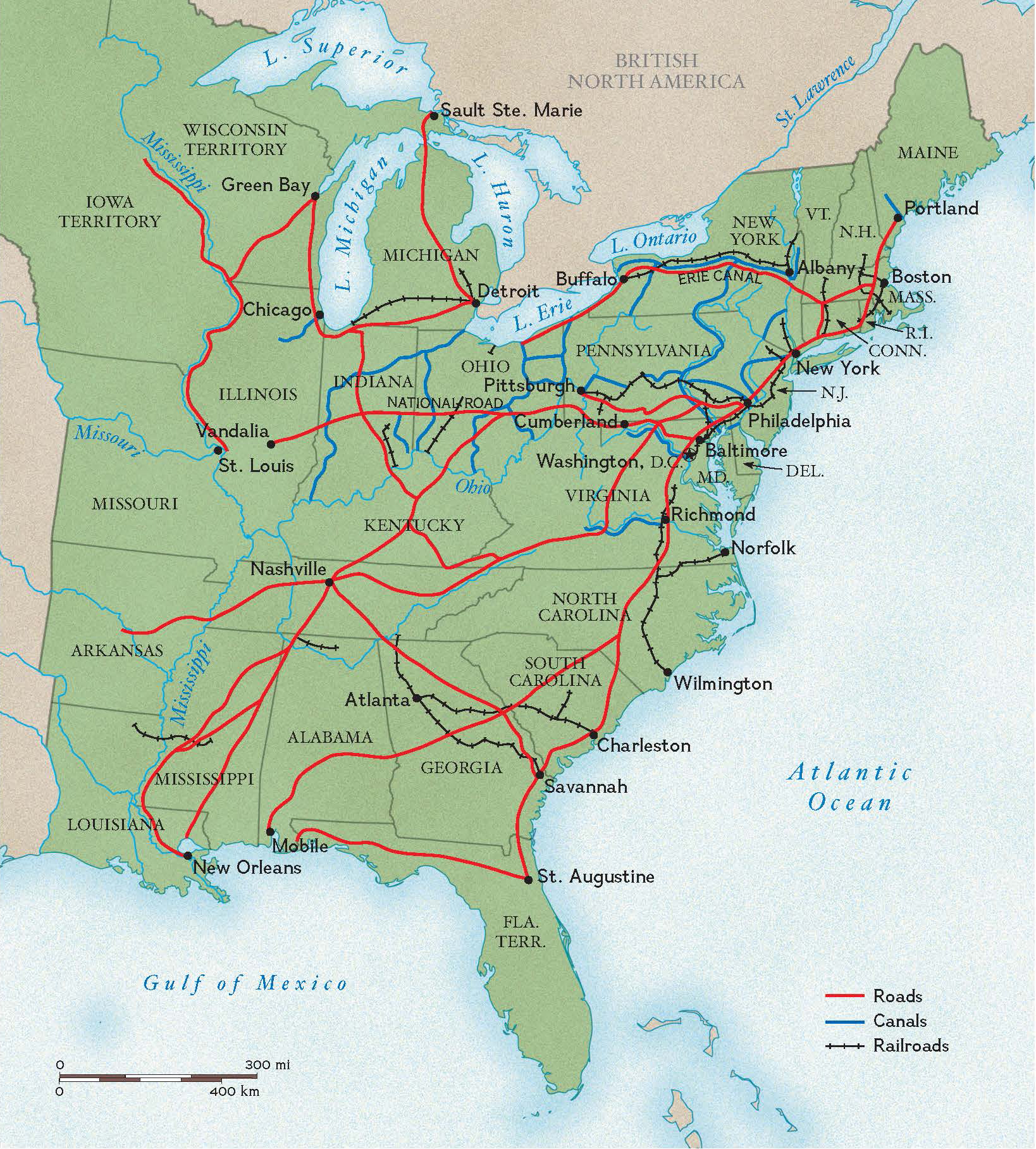The image is a portrait-oriented map of the eastern half of the United States. Dominated by a light green coloring to denote individual states, the map covers from Iowa, Missouri, Arkansas, and Louisiana to the eastern seaboard. Notably, states to the left of Iowa, Missouri, and Arkansas are slightly visible in a tan brown hue, while Canada appears in a brown color. The five Great Lakes are prominently marked in blue, with significant detail on Michigan's rivers. The Atlantic Ocean and Gulf of Mexico, tinted in blue, frame the map along the bottom and right edges. An intricate network of transportation routes is represented: red lines for roads, blue lines for canals, and black lines for railroads. This detailed map offers a comprehensive glimpse of the transportation infrastructure in the eastern United States.